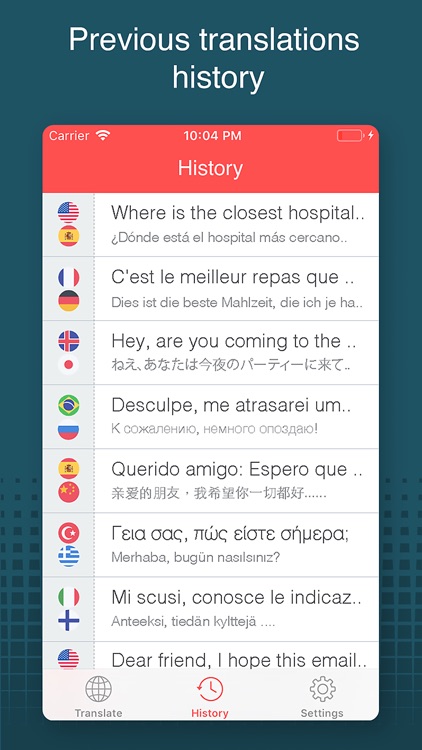A screenshot of a mobile phone displaying the "Previous Translations History" page against a blue background with white text. The device status bar shows it is connected to a carrier and Wi-Fi, with the time displayed as 10:04 p.m. The screen lists various translations, with partial excerpts visible:

1. "Where is the closest hospital...?" with a translation underneath.
2. "Sys lab muller rupes k..." (Note: 'Meilleur' is incorrectly spelled as 'm-e-i-l-l-e-u-r').
3. "Hey, are you coming to the..." with 'discouple discoupe me a traceret...' as the translation. It includes the misspelled 'a-t-r-a-s-a-r-e-i'.
4. "Credo amigo espero k..." with the proper spelling 'q-u-e-r-i-d-o' for 'querido'. A translation is shown underneath.
5. Two more translations follow, with the third one partially cut off, making the total number unclear.